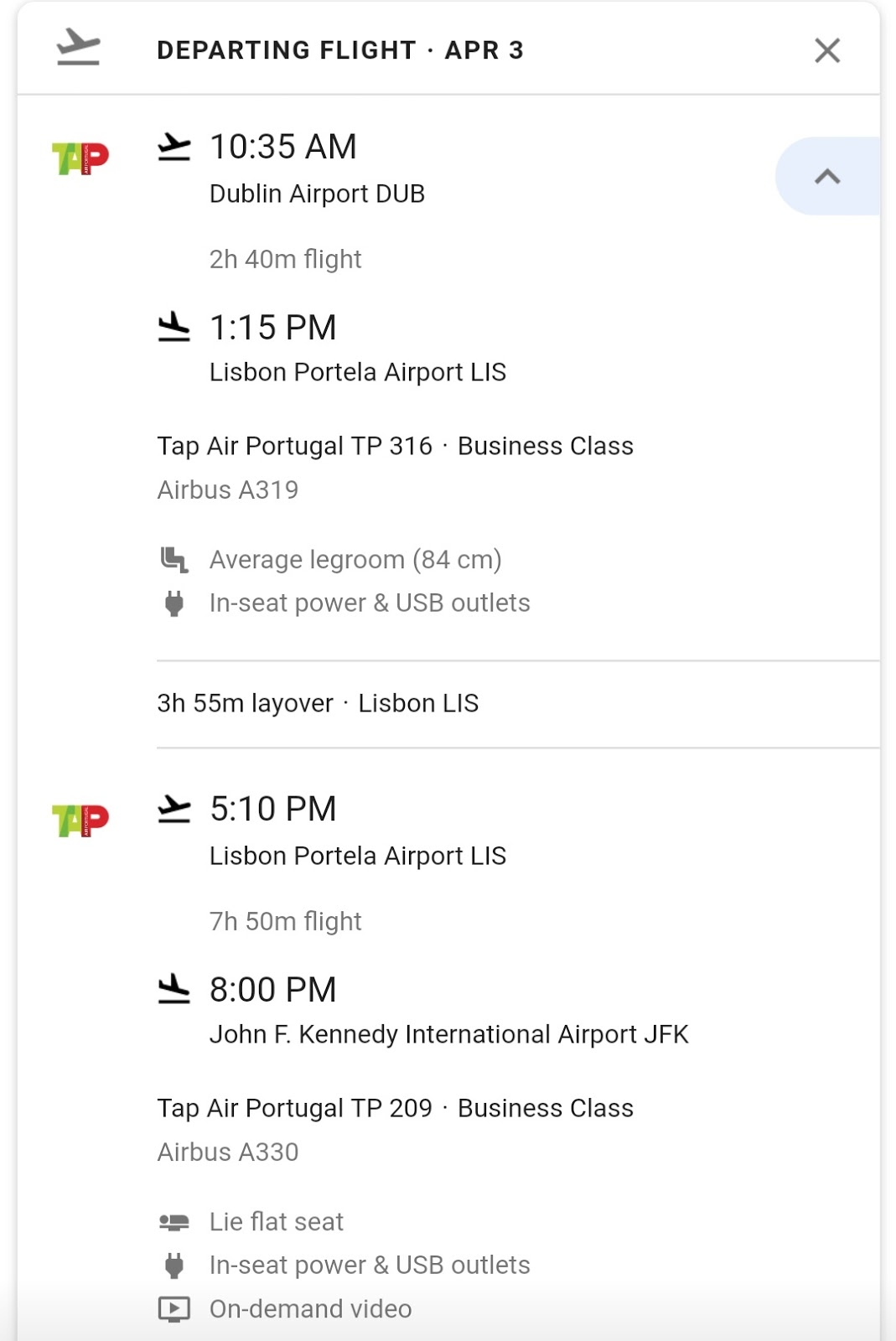This is a detailed screenshot of a departing flight itinerary scheduled for April 3rd. The screenshot is divided into two sections, each marked with a TAP icon on the left.

The first section details a flight departing at 10:35 a.m. from Dublin Airport in Dublin. This flight, operated on an Airbus A319, has a duration of approximately 2 hours and 40 minutes and is scheduled to land at 1:15 p.m. in Lisbon, Portela Airport in Portugal. Adjacent to the departure and arrival times are icons of an airplane: a plane tilted upward for the departure and a plane tilted downward for the landing.

Following this, the itinerary includes a layover in Lisbon lasting 3 hours and 55 minutes.

The second section outlines the subsequent flight departing from Lisbon at 5:10 p.m. This flight is bound for John F. Kennedy International Airport in New York and is expected to land at 8:00 p.m. This leg of the journey is on a business class Airbus A330, which boasts features such as lie-flat seats, in-seat power and USB outlets, and on-demand video. Similar to the first section, this part of the itinerary also uses airplane icons to indicate departure and arrival statuses.